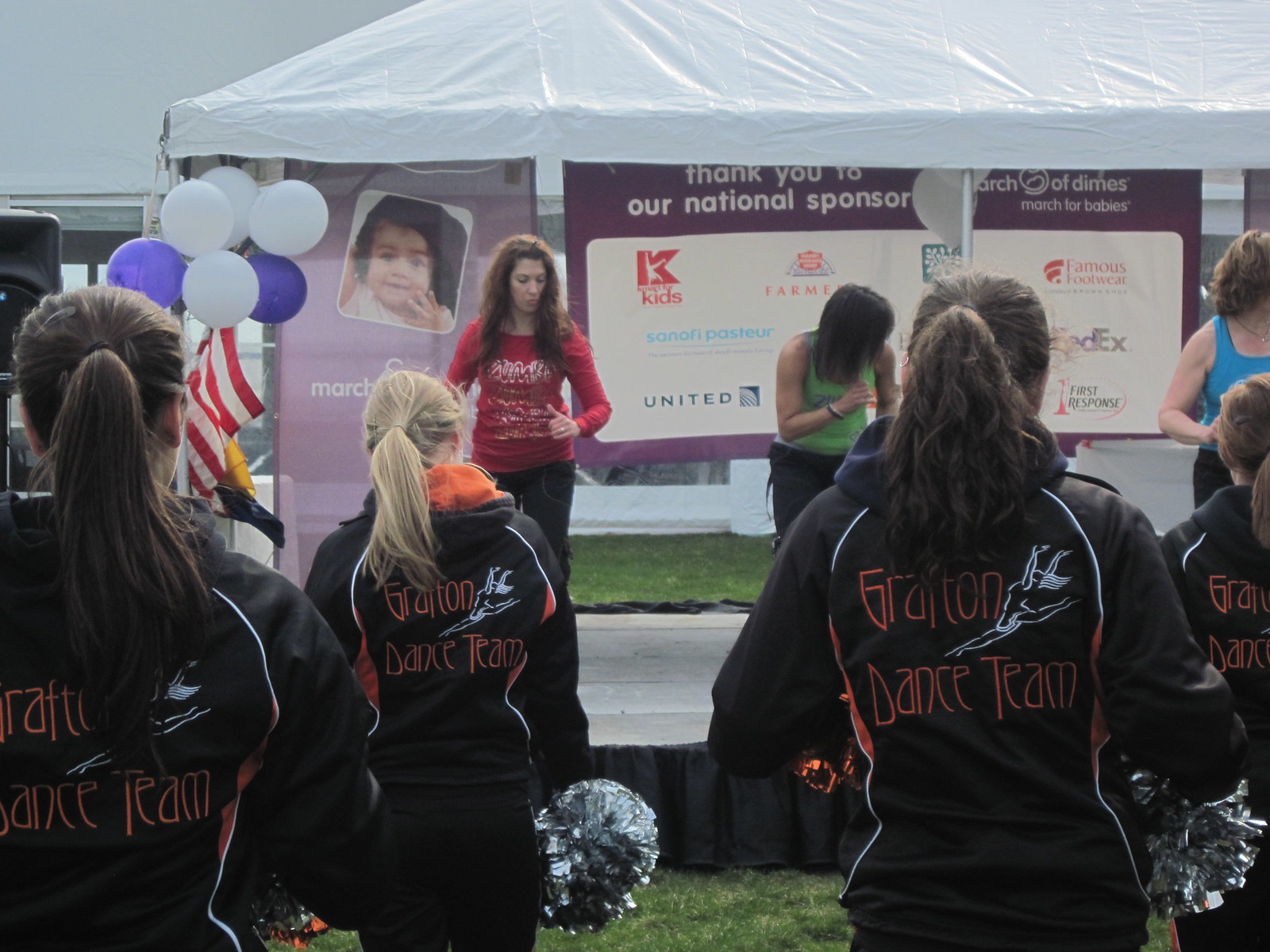This outdoor image captures an event featuring the Grafton Dance Team and what appears to be a March of Dimes fundraiser. The scene is set under a canopy adorned with blue, white, and purple balloons, and an American flag on the left side. On the stage, there are three women, each dressed in distinct colors—red, green, and blue—executing dance moves. Behind them, signage reads, "Thank you to our national sponsor March of Dimes," alongside a poster of a child and logos from sponsors like United Airlines and FedEx. Facing the stage, with their backs to the camera, is the Grafton Dance Team in matching black outfits and jackets emblazoned with "Grafton Dance Team." They are holding silver pom-poms, ready to perform or cheer in support of the event.